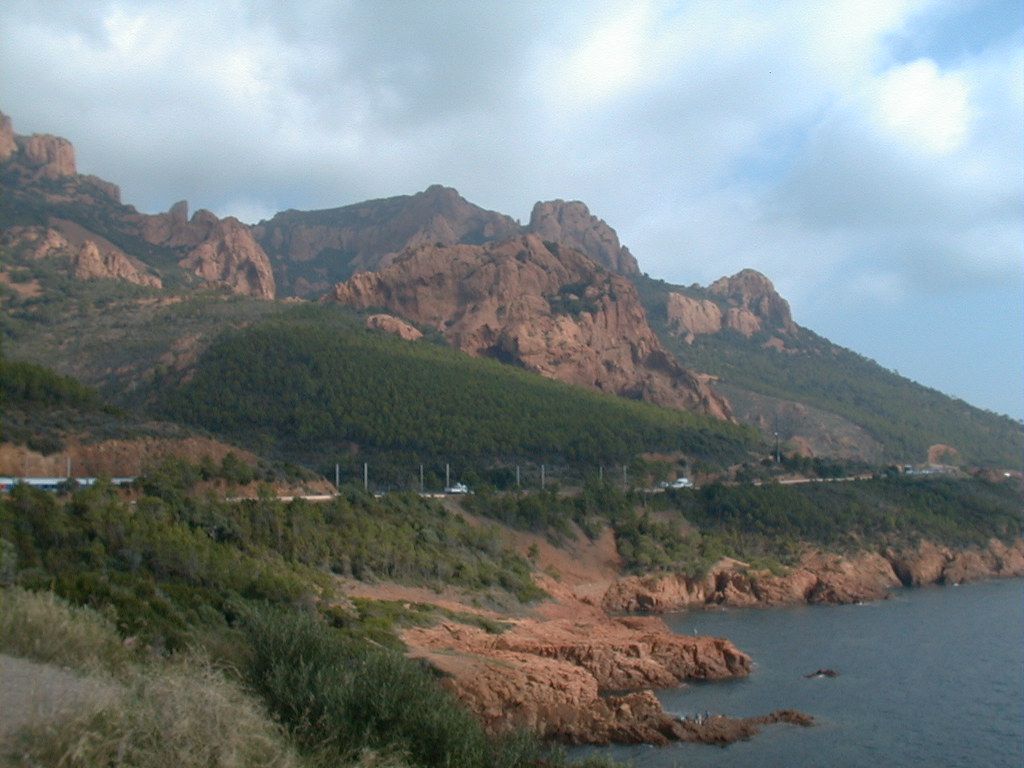This full-color photograph, captured outdoors on a cloudy day, showcases a diverse and vibrant landscape dominated by thick cumulus clouds at the top. Between the clouds and the ground, rugged, brown rocky cliffs and mountains are visible, their bases shrouded in green vegetation. The middle of the image features a road dotted with several cars, including white ones, all traveling towards the left. The road is lined with fence poles for safety. Below this, the landscape slopes down to meet the rocky, scrub-brush-covered shore of a serene body of blue water. The foreground is a mix of green rolling hills and bushy grass, adding layers of texture to the scene, while the background climaxes with additional green hills and majestic mountains.